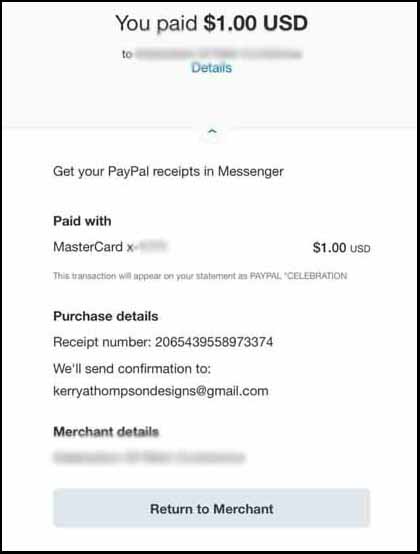The image depicts a PayPal payment receipt displayed on a screen. The receipt is enclosed in a small rectangle with a black border. At the top of the screen, it indicates that a payment of one US dollar has been made, but the recipient's details are obscured by a faded line for privacy. Below this is a "Details" hyperlink.

Further down, there's a heading that reads "Get your PayPal receipts in Messenger." It specifies that the payment was made using a MasterCard, though only the last four digits of the card are hidden. The amount paid is clearly shown: one US dollar.

Following this, another heading states "Purchase Details," displaying a receipt number: 206-543-955-897-3374. It also mentions that a confirmation email will be sent to kerry@thompsondesigns@gmail.com. The merchant details are again obfuscated, ensuring privacy.

At the very bottom of the image is a grey button with black text that reads "Return to Merchant."